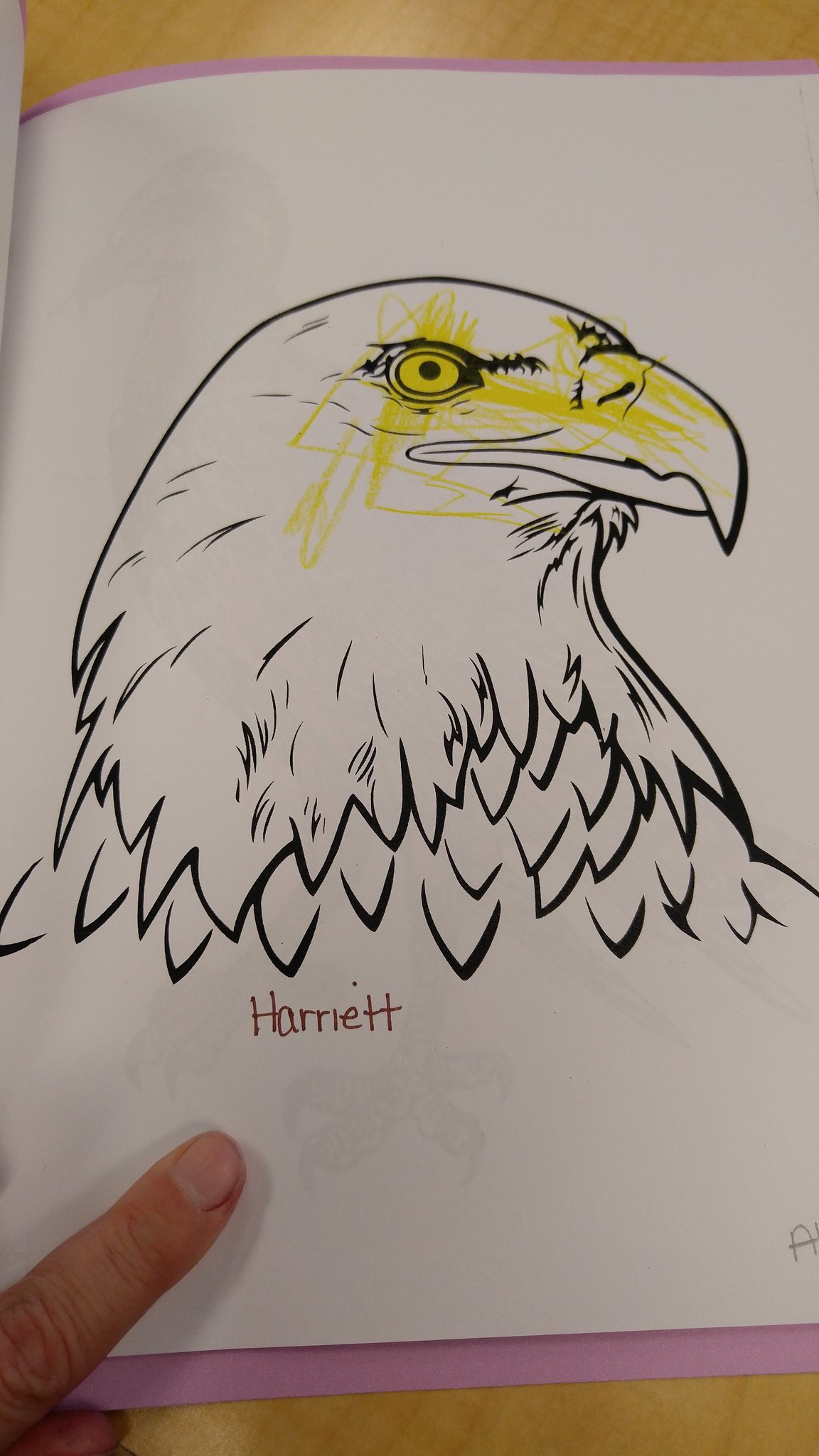This image showcases a black and white line drawing of an eagle's head, reminiscent of a coloring book illustration. The drawing is predominantly uncolored, except for a splash of yellow marker artfully and somewhat messily applied over the eagle's eye, beak, and part of its head, suggesting the handiwork of a child. At the bottom of the eagle's head, the name "Harriet" is written in thick brown marker, with the letters spaced out as "H A R R I E T T." The white page featuring this artwork is placed on top of a purple paper, with the purple color visible at the top and bottom edges. In the left-hand corner, a finger points towards the name "Harriet," casting a faint shadow on the page beneath it. In the right-hand corner, the letter "A" is partially visible, hinting at another word or name that isn't fully shown. The entire setup rests on a brown wooden table, adding a natural texture to the background.